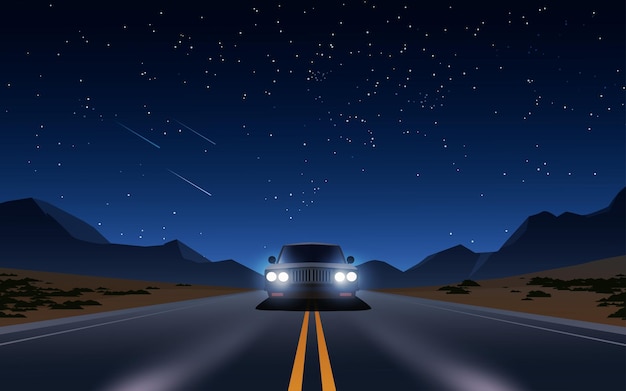The image appears to be a computer-generated or video game graphic depicting a nighttime scene with a sense of depth and perspective. The dark blue sky, transitioning to lighter hues near the horizon, is sprinkled with numerous white stars, and towards the left, three shooting stars streak towards the ground. Dominating the scene is a solitary car driving directly over the double yellow lines of a road that stretches from the foreground into the distance. The car's headlights are on, illuminating the immediate area, suggesting nightfall. Blacked-out windows obscure the inside of the car. Surrounding the road are patches of dirt and grass, while mountain ranges frame the image on both the left and right sides, adding to the overall dramatic and atmospheric composition.